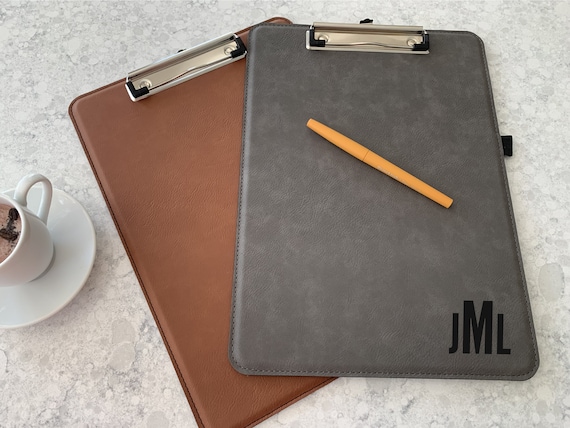The photograph depicts two clipboards with a leather-like, cushioned vinyl binding. The clipboards are positioned on a predominantly white marbled counter with grayish circular streaks. The brown clipboard lies at a diagonal angle, while the gray clipboard, positioned on top, sits more straight. The gray clipboard features a logo with the initials "JML" in capital letters, with the "M" taller than the "J" and "L," located on the lower left corner. A yellow pen is angled across the gray clipboard, running from around the 10 to 4 o'clock positions. A possible pen loop is also visible on the right side of the gray clipboard. To the left of the clipboards is a white mug on a white saucer, which appears to contain a cappuccino with some form of cream. This cup stands out against the marble countertop, adding a touch of warmth to the scene. The gray clipboard and the brown clipboard both have silver clips at the top.